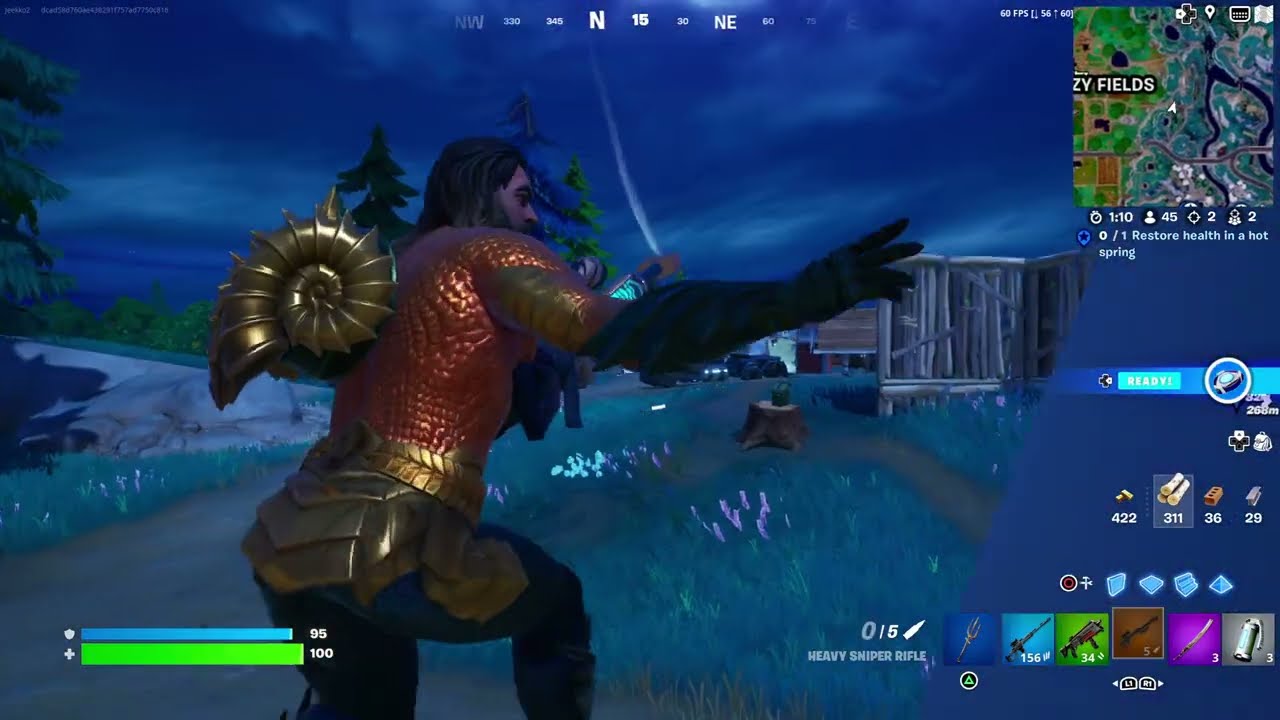This screenshot from the video game Fortnite features the character Aquaman, highlighted by his gold sequined suit, green gloves, and green pants. He is prominently positioned slightly left of center, outdoors in a dark, possibly night-time setting. On his back, he wears a conch shell that may be a jet pack. The scene around him includes buildings, pathways, green grass, trees, rocks, and stumps, with a shed visible in the background and possibly a small body of water in the upper right. The HUD displays various in-game elements such as the compass, map, player health, weapons, and tools, accentuating the colorful in-game environment with blue, green, orange, gold, black, purple, gray, and white hues. Text on the screen includes objectives like "restore health in a hot spring." Aquaman appears to be in an action pose, possibly throwing or catching something with his right hand.